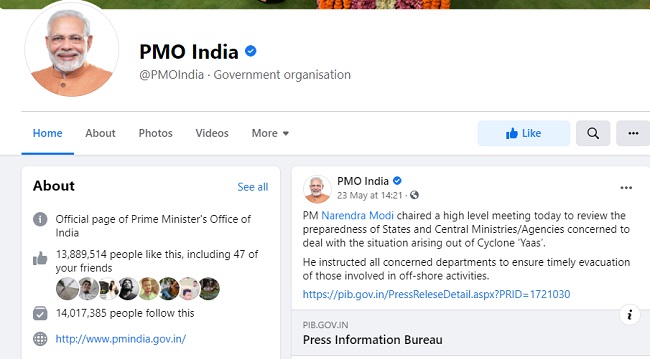The image depicts a Facebook page that mirrors the typical layout of the social media platform, complete with recognizable fonts and features. At the top, a prominently displayed profile picture of a man suggests the identity of the page owner. Adjacent to the image, the text reads "PMO India," identifying the page as that of the Prime Minister's Office of India under the category "Government Organization." 

Directly beneath this, the standard Facebook navigation headings "Home," "About," "Photos," "Videos," and "More" are listed, suggesting where users can find additional content. On the right side, a "Like" button, a search bar, and an options menu represented by three dots are available for user interaction.

On the left, an "About" section details the number of friends and followers, with a clickable "See All" link for further details. The right side features the page's latest post from "PMO India," providing new information and a website link for more details. Below this post, there's an information bar labeled "Press Information Bureau," accompanied by an icon of a circle containing an 'i', signaling the availability of additional information.